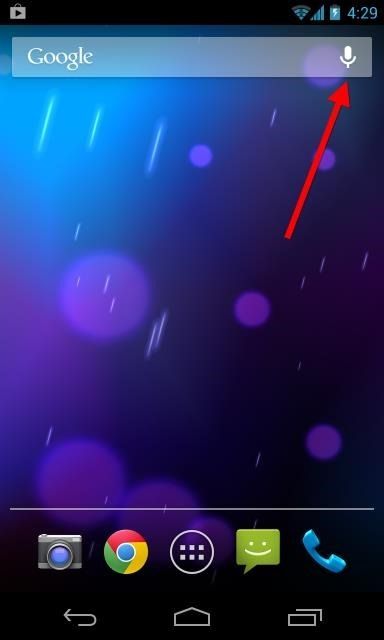An image depicting a Google home screen reveals a minimalistic background with a muted, rain-like aesthetic interspersed with purple orbs. Dominating the top part of the screen is a black status bar featuring various icons: a Google Play Store icon on the top left, signal strength with four full bars, and a nearly full battery icon at around 90%. Adjacent to these on the right, the current time is displayed in blue numerals (4:29 PM) next to an upward-pointing arrow and a microphone icon.

Centrally positioned at the top is the Google search bar, identifiable by the Google logo on the left. Below the search bar are four primary app icons: a camera on the far left, Google Chrome next to it, an app drawer icon (a circle with four squares) at the center, and a messaging app with a green text bubble icon on the far right. At the bottom-most part of the screen lies a horizontal block containing navigation icons for back, home, and task view functions.

Overall, the screen presents a clean, user-friendly interface typical of Google's design philosophy.